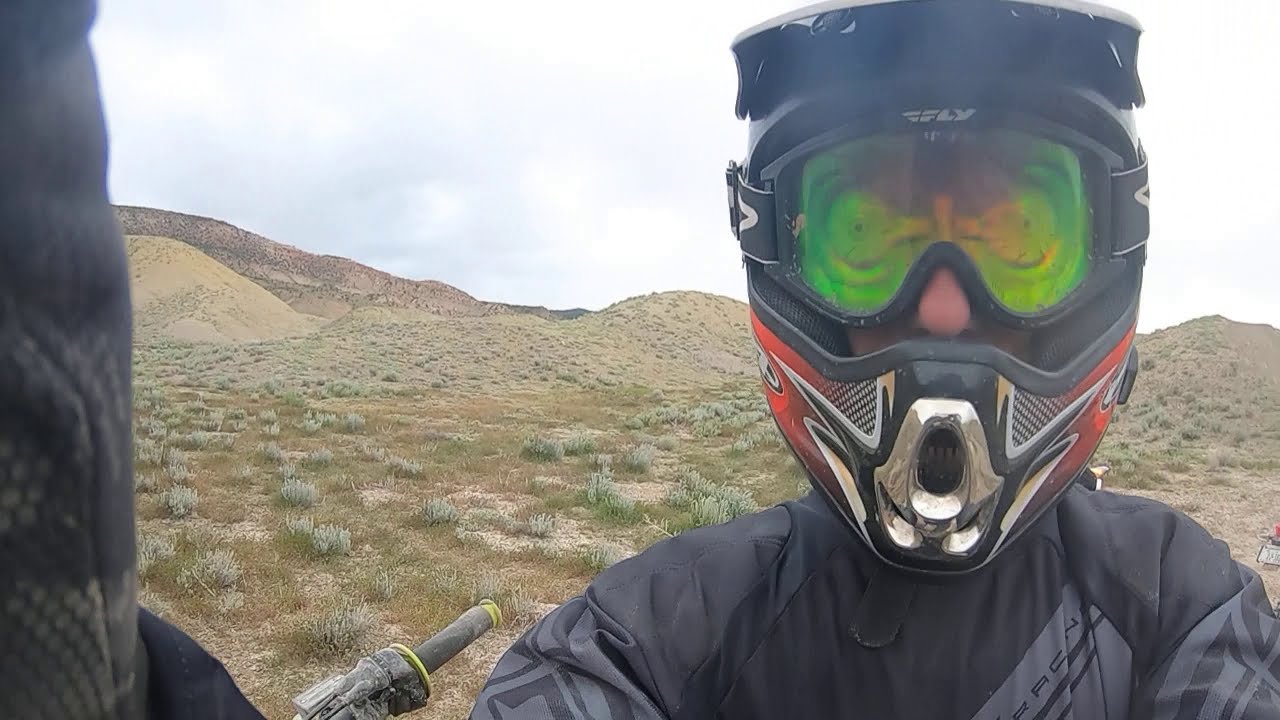In this captivating image, a motorcyclist in a desert landscape captures a selfie, giving us a front-facing view of their striking gear and the surrounding scenery. The rider wears a full protective helmet adorned with bright green goggles, which transition to orange in the middle and feature a distinctive black smudge. The helmet itself is detailed with a black plastic ridge on top and a noticeable silver-colored circular breathing port at the bottom, flanked by black streaks outlined in silver. The figure is dressed in a black long-sleeve motorcycle jacket, and on the far left edge of the image, the elbow patch of another person is visible. A dirty black handlebar with a green outer spot and a green inner ring is seen to the left and bottom of the rider, hinting at either a motocross or mountain bike. The landscape behind them consists of rolling sandy hills with patches of green grass and white flowers, resembling a rugged desert terrain ideal for off-road biking. The overcast sky above is a mix of gray and white clouds, adding a dramatic backdrop to this adventurous scene.